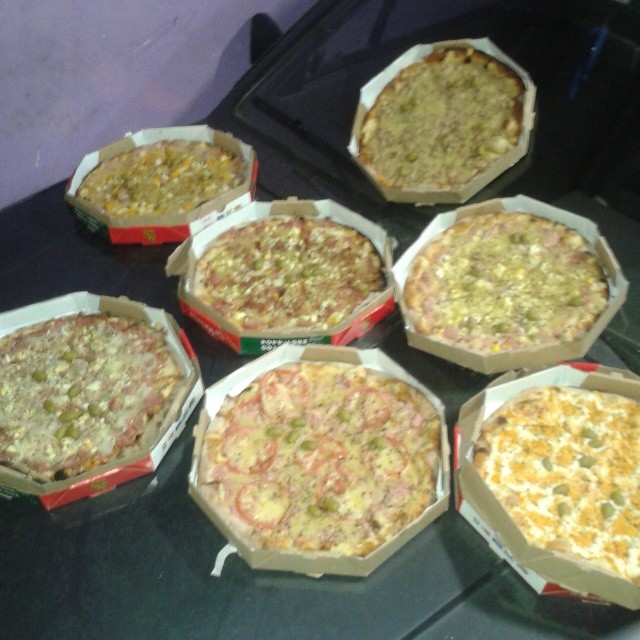This overhead photographic image captures seven gourmet, personal-sized pizzas, beautifully arranged in the center of the frame. The pizzas are collectively presented without lids, nestled in uniquely shaped cardboard boxes that resemble octagons. The vibrant boxes feature red, green, and white colors on their sides, enhancing the visual appeal of the scene. The pizzas are thoughtfully positioned: three on the right, two in the middle, and two on the left. Each pizza boasts an array of intricate toppings, showcasing diverse flavors—from green olives, tomatoes, and cheese to sausage, pepperoni, and perhaps ham or bacon. The pizzas rest atop a black car, adding an unexpected backdrop element to the image. The overall composition emphasizes the colorful and appetizing variety of the pizzas, making them the focal point of the photograph.